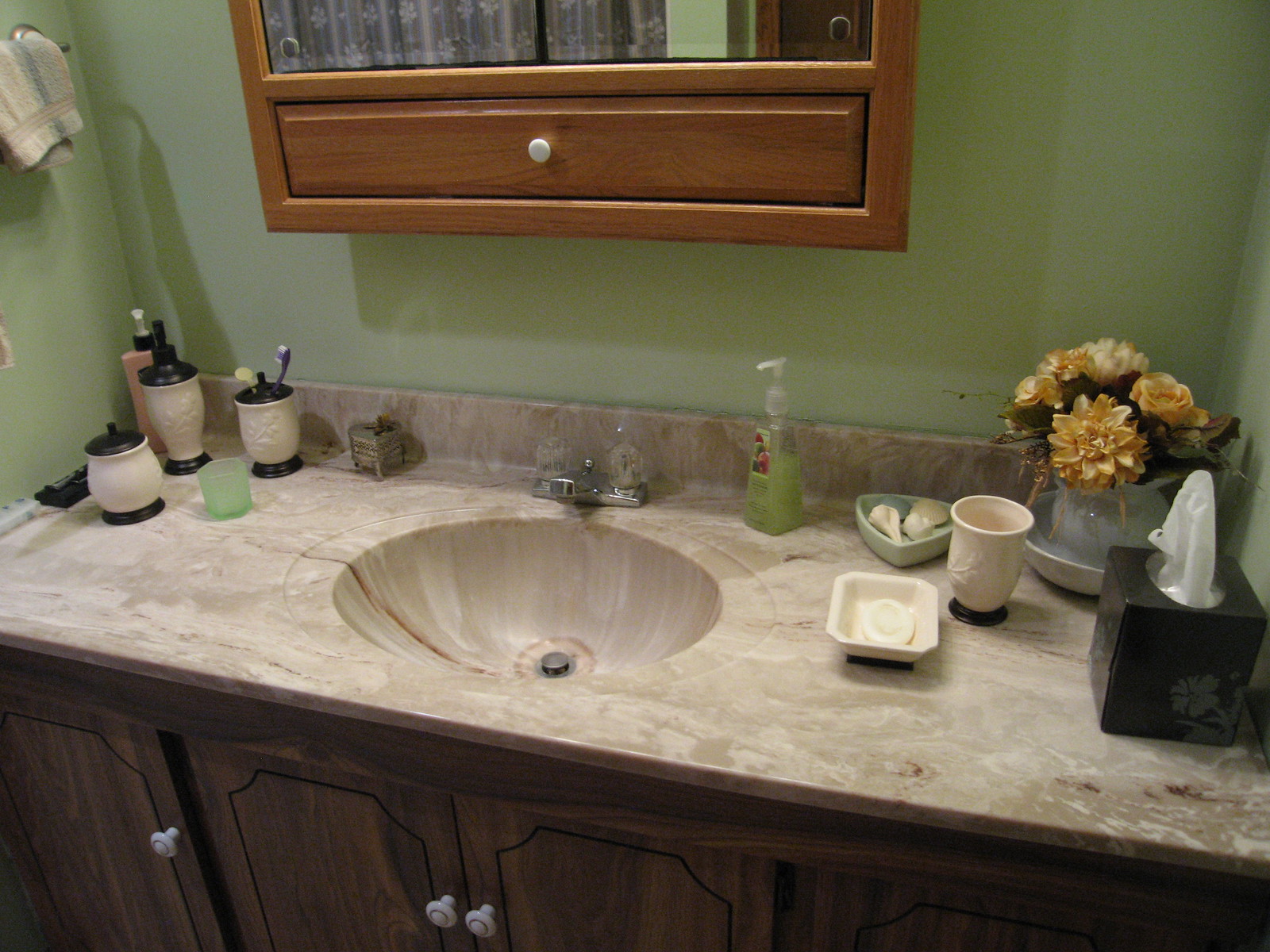The image captures a neatly organized bathroom countertop and the wall behind it, presenting a snapshot of a well-decorated and meticulously maintained space. The wall features a light green paint, imparting a calming ambiance to the room. On the upper left side of the photograph, a white towel with a blue gradient hangs gracefully from a silver towel rod. 

At the center of the image, a light brown cabinet with a white knob takes a prominent position. The adjacent mirror, though partly cut off, hints at the reflection of the well-appointed room. Below the countertop, medium brown cabinets adorn the scene, uniformly equipped with white knobs, providing both storage and visual balance.

The countertop itself is an elegant expanse of tan marble, infused with intricate veins of darker brown and white. This beautiful marble surface extends seamlessly into the sink basin, enhancing the cohesive design of the bathroom. The silver metal faucet, accompanied by clear glass dials, adds a touch of modernity to the classic decor.

To the left of the sink, a trio of white ceramic canisters with black bases and floral prints provide stylish storage. One canister holds an array of toothbrushes, while another houses a soap dispenser. A clear hand soap dispenser containing green soap is positioned to the right, reflecting the room's color scheme. 

Further to the right, a black tissue box adorned with a gray flower design ensures tissues are readily available. A white ceramic vase filled with vibrant yellow flowers completes the scene, adding a cheerful splash of color and a touch of nature to the space.